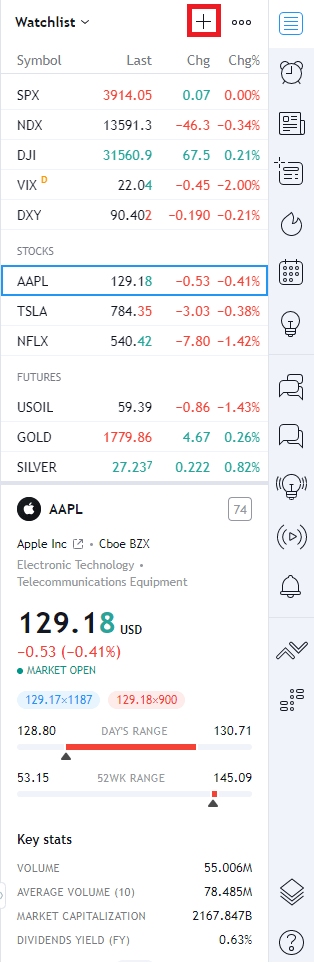The image is a detailed screen capture of a stock watchlist interface. It's a long and narrow display primarily showcasing various companies' stock tickers and their daily activity. At the very top, the header is labeled "Watchlist," followed by a prominently highlighted red box around an "Add" button, suggesting the option to include more stocks to the watchlist.

On the right edge of the screen, a vertical array of icons extends from top to bottom, including symbols for an Alarm Clock, News, Breaking News, Trends, Calendar, and Messages among others. These icons likely offer quick access to related functionalities or information.

The main portion of the image is dedicated to the stock tickers and their daily performance metrics, categorized into four distinct columns: Symbol, Last (representing the last traded price), Change, and Change Percent. The stock symbols listed include major indices like SPX, NDX, DJI, VIX, and DXY, as well as individual stocks such as AAPL (Apple), TSLA (Tesla), and NFLX (Netflix). There is also a Futures section that includes commodities like USOIL (crude oil), Gold, and Silver. Adjacent to these symbols are their respective numeric values, detailing the last traded price, the absolute change, and the percentage change for the day.

In the bottom middle section of the screen, the stock ticker AAPL (Apple) is specifically selected and highlighted. This area provides comprehensive information about Apple Inc., including its current stock price, the day's performance metrics, and key statistics such as trading volume, market capitalization, and dividend yield. The Apple logo is also displayed prominently alongside this information, offering a quick visual reference.